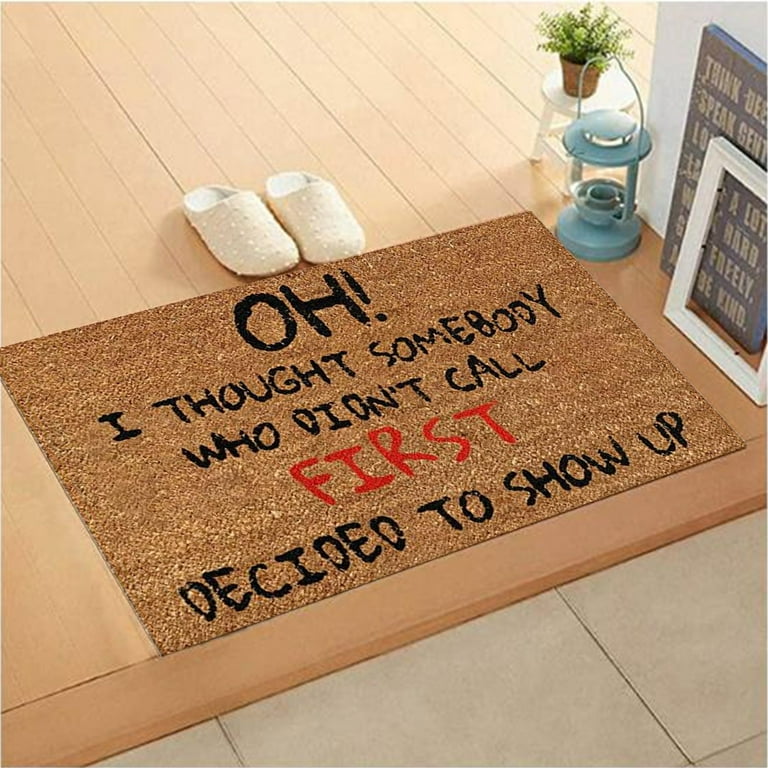This square image showcases a cozy entryway scene with a brown, rectangular outdoor welcome mat prominently displayed at the center. The mat features the playful text, "Oh! I thought somebody who didn't call FIRST decided to show up," with "FIRST" in all caps red text and the rest in black. In front of the mat, there is a pair of white clogs adorned with small dots. To the right, a light blue lantern with a circular base and top, complete with a handle, is positioned nearby. Behind the lantern, a small white stool supports a potted green plant. 

There are two picture frames leaning against the white wall in the upper right corner of the image. The lower right section of the image reveals large, light brown square tiles. Adjacent to the mat, the flooring transitions to a series of diagonally arranged wooden planks. The setting suggests a welcoming yet stylish foyer, blending practicality with a touch of whimsy.